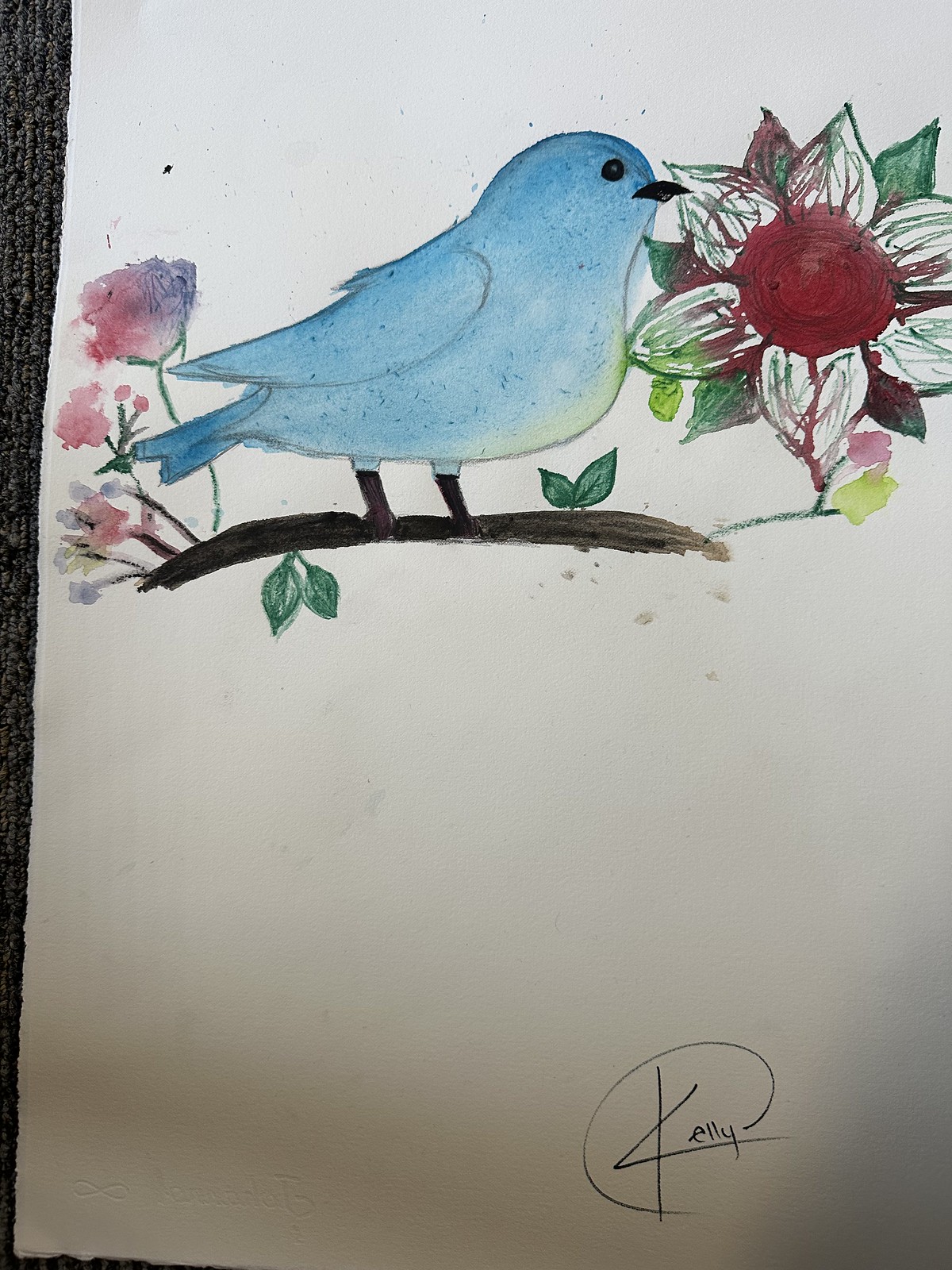A beautifully detailed drawing depicts a serene bird perched on a brown branch with green leaves on a white piece of paper. The bird, rendered with a delicate blend of baby blue and a slight green tint on its belly, adds a gentle charm to the scene. Surrounding the bird are watercolor flowers: to the left, flowers with green stems and a mix of pink and purple petals, while to the right, a striking flower with a red center complemented by white, red, and green leaves. The white paper is bordered on the left by a gray area that appears to be either carpeting or upholstery, adding a subtle texture contrast. The composition is signed by the artist in the bottom right corner: "Kelly."